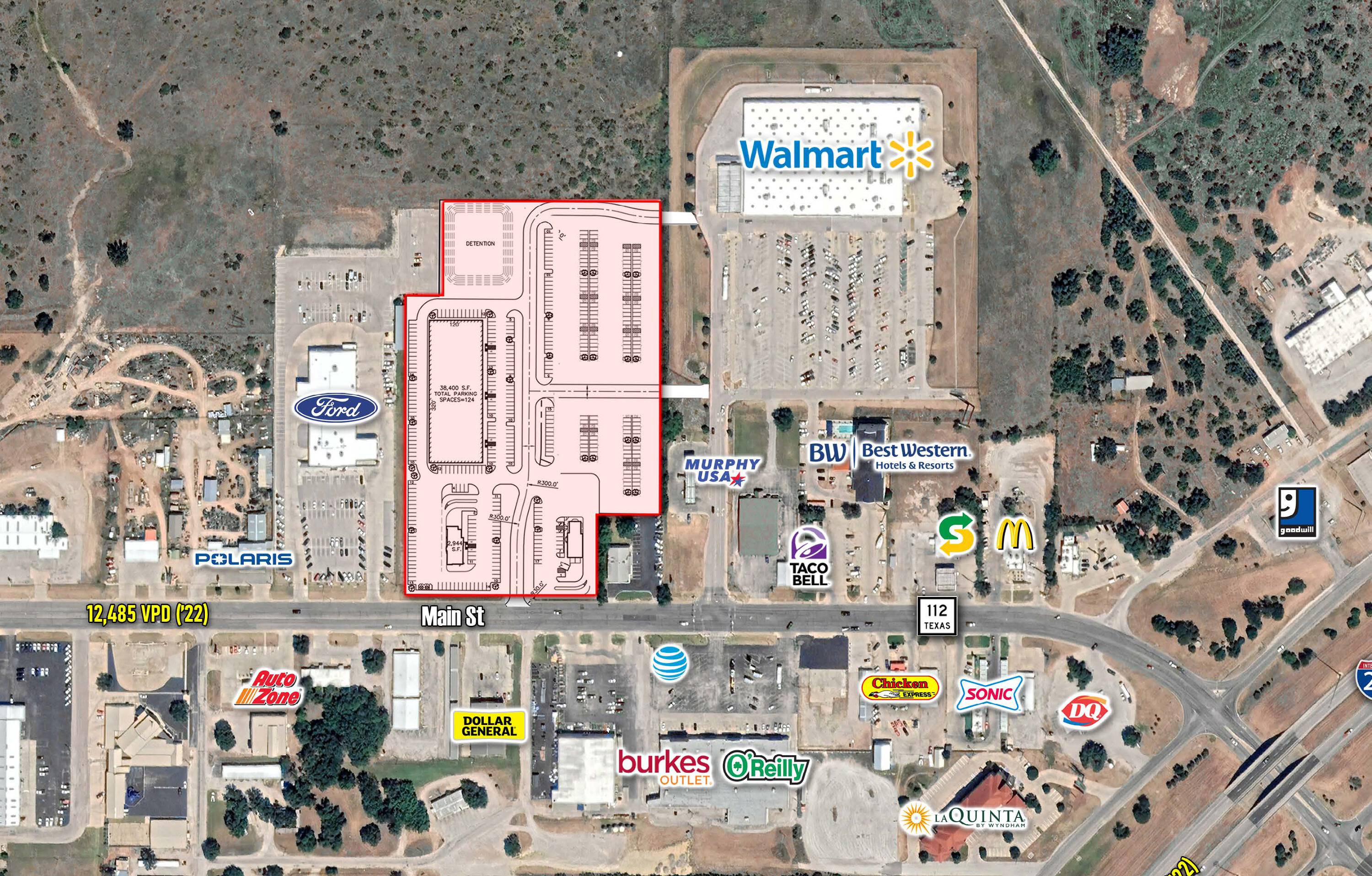This detailed aerial image, possibly from a Google Earth satellite view, showcases a bustling strip in a city, centered around Main Street, also labeled as Route 112 in Texas. The horizontal rectangular image highlights a series of labeled buildings along Main Street, featuring prominent stores and restaurants with recognizable corporate logos atop each building. 

On one side of Main Street, we observe a Walmart with a large parking lot behind it, accompanied by a Murphy USA gas station, Best Western hotel, Taco Bell, Subway, and McDonald’s in sequence. Adjacent to these, there is a Ford dealership next to a field containing sparse green trees. This side also includes a Goodwill and some smaller, unnamed buildings.

On the other side of Main Street, notable establishments include a Dairy Queen, Sonic, a Chicken Place, O’Reilly Auto Parts, Berks Outlet, Dollar General, and AutoZone. Behind the Sonic lies a La Quinta Inn. Further down this busy road, a building marked with an AT&T symbol stands out among additional unnamed buildings.

The roadway network is further illustrated by several unnamed roads branching off diagonally in the bottom right corner of the image. Toward the top edge, beyond the array of commercial buildings, the landscape transitions into a grassy area with scattered trees.

This well-designed, modern map not only emphasizes the density of commercial activity along Main Street but also shows the layout’s integration with the surrounding environment, providing a comprehensive overview of this busy urban strip.